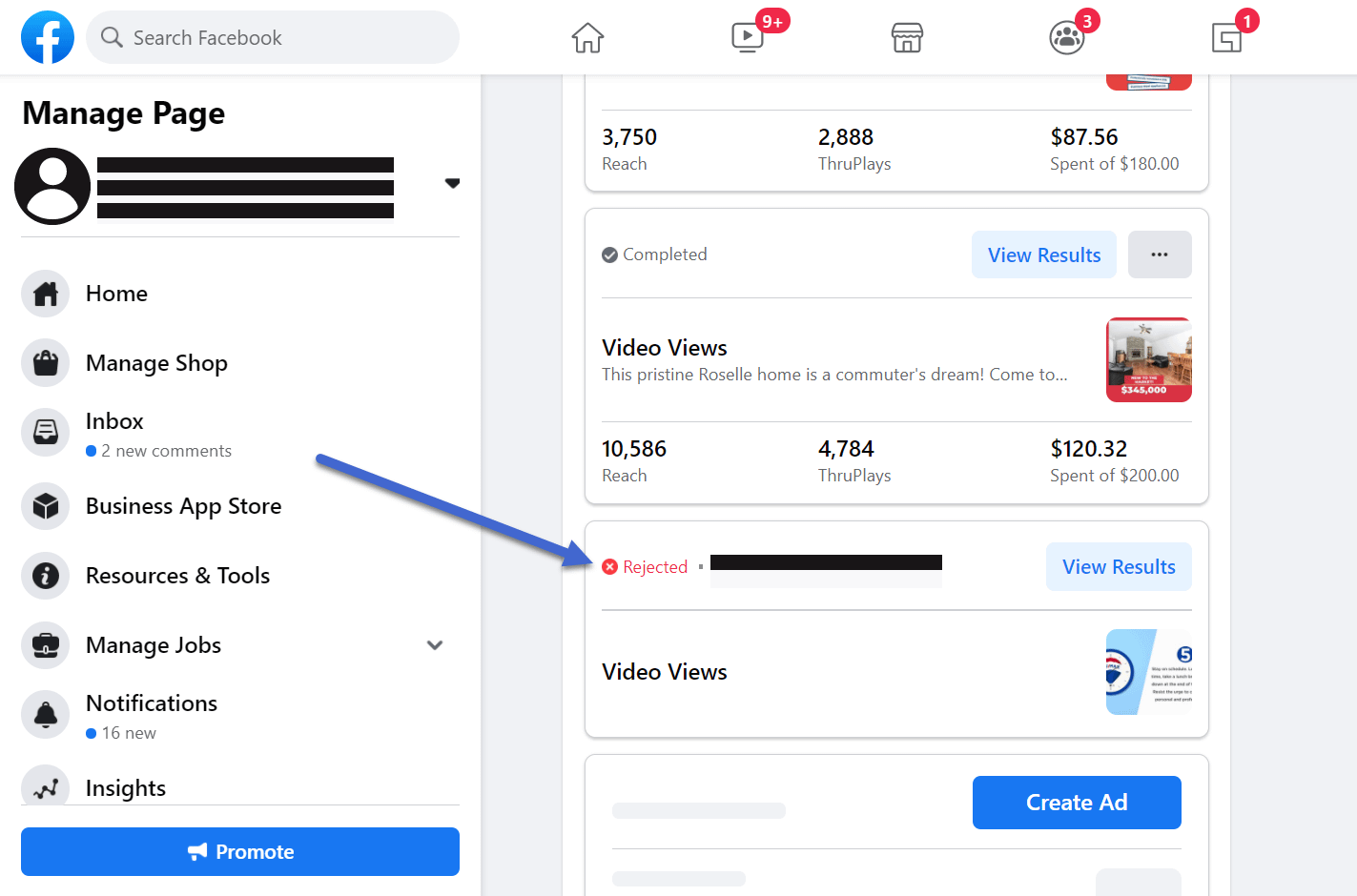**Screenshot of Facebook Business Page Dashboard: Video Rejection Tutorial**

This image captures a detailed screenshot of what appears to be the mobile or desktop view of a Facebook Business Page. The interface shown is indicative of a behind-the-scenes look at the management side of a business account. At the top, familiar Facebook icons are present.

Central to this screenshot is a tutorial-like guide, focusing on the rejection and potential appeal process for content. A prominent red arrow points to the word "Rejected," suggesting the screenshot pertains to how one might handle a video that has been declined by Facebook. Indicators such as "video views" and "results" above the rejection suggest the rejected content is indeed a video.

On the left sidebar, a range of management tools and resources are visible including: Home, Manage Shop, Inbox, Business App Store, Resources and Tools, Management Jobs, Notifications, and Insights. Additional actionable buttons like "Promote" and "Create Ad" are prominently displayed, allowing quick access to advertising functionalities.

The image also reveals analytical data about video performance, such as views and expenditures, giving a snapshot of how various videos are performing financially. Altogether, the dashboard provides a comprehensive suite of tools for managing videos and advertisements, likely catering to a business, brand, or creator.